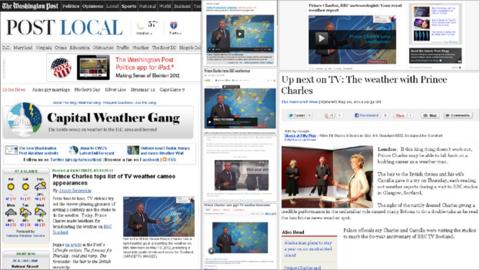The image depicts a webpage from the Washington Post's website. At the very top, the iconic "Washington Post" logo is prominently displayed against a black navigation bar that lists different sections of the site. Just below this bar, the "Post Local" section is visible, accompanied by various symbols.

Further down the page, there is a featured news story, which is followed by a segment titled "Capital Weather Gang." This segment includes a graphic featuring the Capitol building and a storm cloud, symbolizing weather-related content. Adjacent to this image, additional graphics depict the sun and clouds, among other weather icons.

On the right-hand side of the page, there is a mention of Prince Charles, suggesting a list of upcoming TV weather appearances. Along the left side of the page, several videos of weather presenters are displayed. At the far left, another segment titled "Up Next on TV" highlights the weather report by Prince Charles. Below this, there are multiple images of television presenters, accompanied by descriptive text.

Overall, the webpage serves as a comprehensive hub for various news stories and weather updates, featuring a blend of text, images, and multimedia content from the Washington Post.